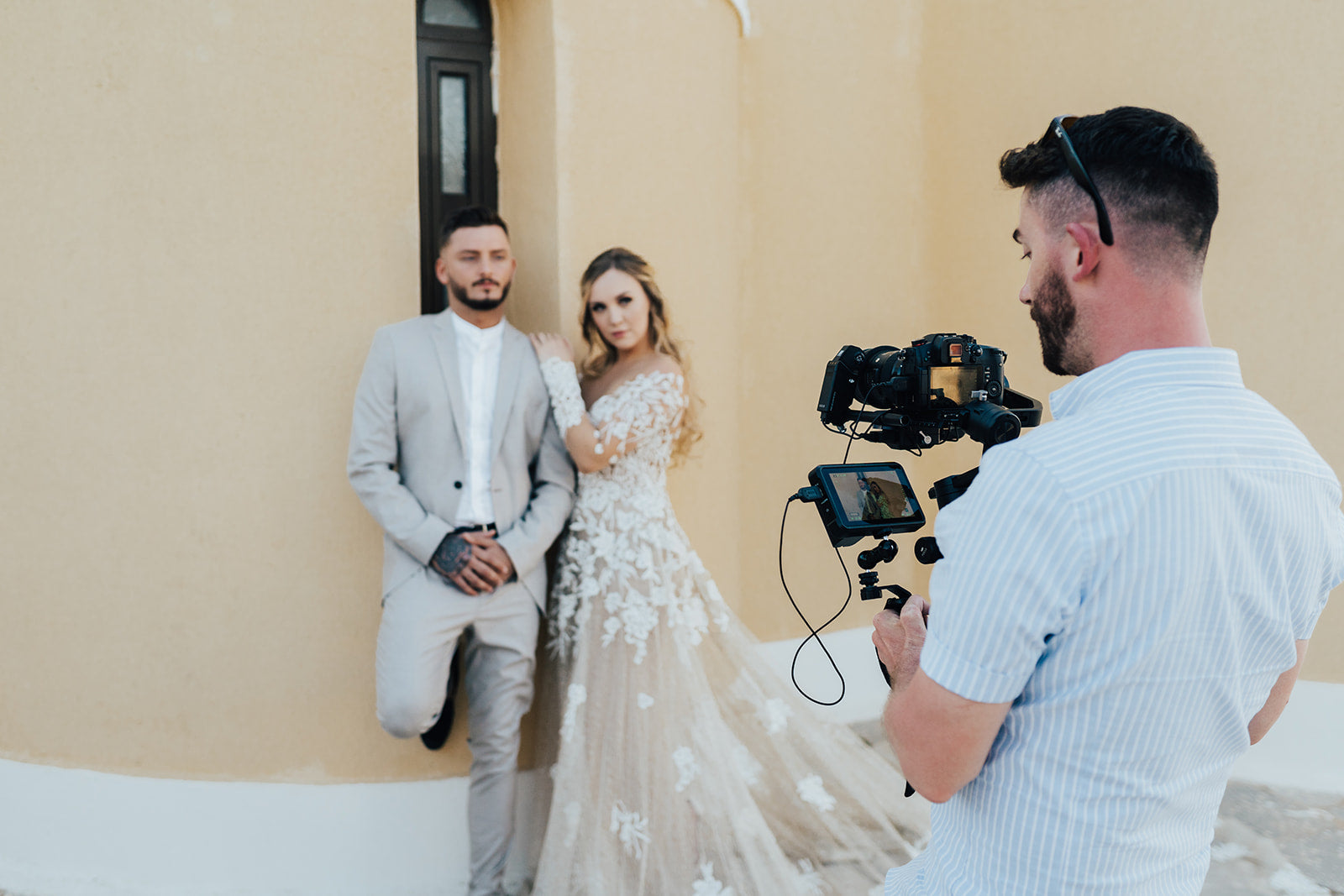In this captivating and detailed wedding photograph, we observe a photographer from behind, capturing a memorable moment for a bride and groom. The photographer has short brown hair, a beard, and wears sunglasses on the top of his head. Dressed in a short-sleeved, light blue, and white striped shirt, he carefully looks through the viewfinder of his camera while holding a screen. The couple stands against a light yellow or sherbet orange wall with a white base, featuring a small frosted window with a black frame in the background.

The bride, standing to the right, is a Caucasian woman with long blonde hair that has brown highlights at the top. She stuns in a lace-covered wedding dress that is transparent in parts, flaring out elegantly into tulle at the bottom. Her arm is affectionately resting on the groom's shoulder. The groom, with brown hair, is sharp in a light gray suit paired with a white shirt. He casually leans against the wall, his right foot propped up and his right hand revealing a tattoo. The harmonious arrangement and intricate details make this image a beautiful representation of their special day.